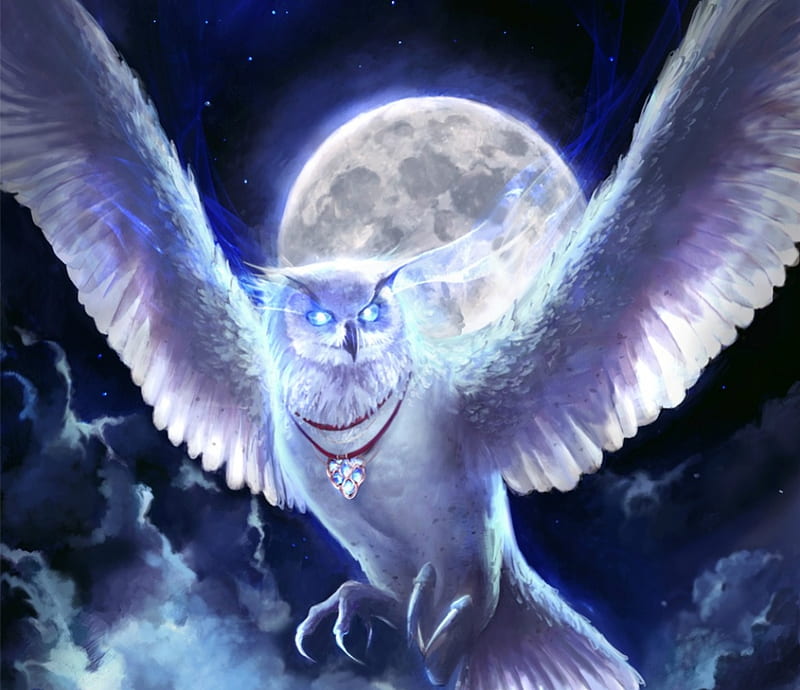In this digital artwork set against a deep blue night sky sprinkled with stars, a white owl dominates the scene as it soars with its wings spread out and upwards. The owl’s head, which appears slightly small for its body and is turned slightly to the right, exudes an almost fantastical quality. Its eyes gleam like bright gemstones, adding a mystical touch. Adorned around the owl's neck are two red necklaces, one simple and one featuring a cluster of gemstones. The moon behind the owl casts a bluish glow, surrounded by a faint halo of lighter purple, illuminating the surrounding clouds which are a mix of whitish and dark black hues. Adding to the mythical ambiance, wisps of smoke trail from the owl’s ears, blending into the night sky. The scene strikes a balance between serenity and surrealism, crafting an enchanting nocturnal fantasy.